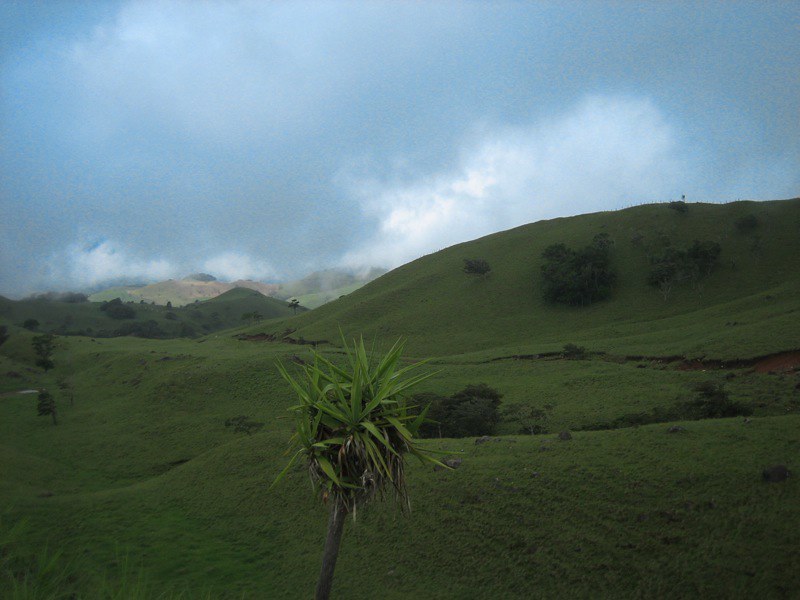This vibrant outdoor photograph captures a vast, lush landscape under an overcast sky. The foreground features a prominent plant with a grayish-brown trunk and spiky green leaves, possibly a weed, standing amid rich green grass and dense vegetation. This central plant is surrounded by a beautifully textured field of rolling hills covered in thick, vivid green grass, with sporadically placed darker green bushes and shrubs. The mid-ground reveals a grassy depression and a dark road at the base of rolling hills, leading to distant gray mountains shrouded in rain or mist. The sky, dominating the top half of the image, is heavily clouded, with white clouds hanging low and some sunlight breaking through to cast a subtle glow over the landscape. The entire scene is devoid of any text, emphasizing the natural beauty of the setting.